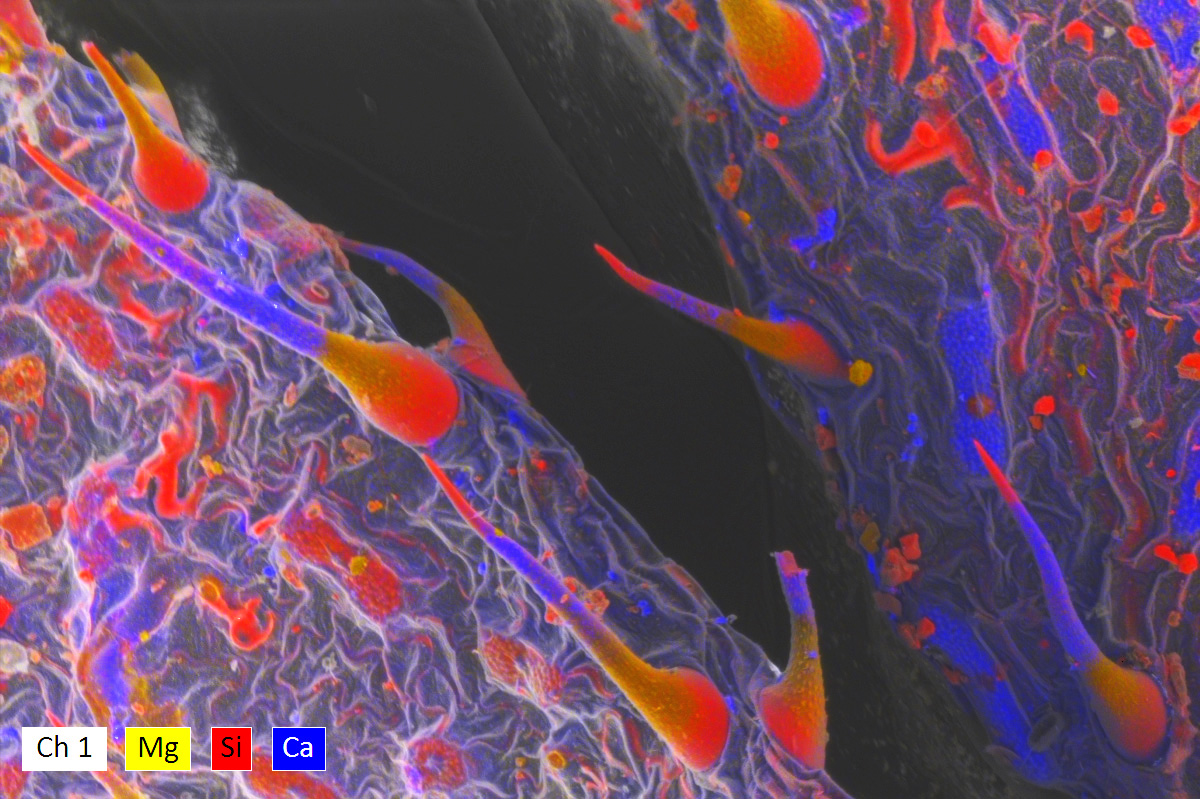The image on the computer screen appears to be a highly magnified, color-coded microscopic photograph, potentially from a scientific textbook. The image displays what seem to be blood vessels or arteries, illuminated in striking neon colors including shades of red, blue, orange, yellow, and purple. These vibrant colors may indicate different mineral compositions or elements. Emerging from these vessels or fibers, which resemble thick hair follicles, are various colors transitioning from bright orange at the base, through yellow and blue, to a reddish tip. The photograph is divided into sections with each color representing a different element: CH1 in white text with a black border, MG in a yellow box, SI in a red box, and CA in a blue box. Additionally, there is a large black area dividing the sample into two distinct sections, further suggesting a detailed scientific study of the elements involved.